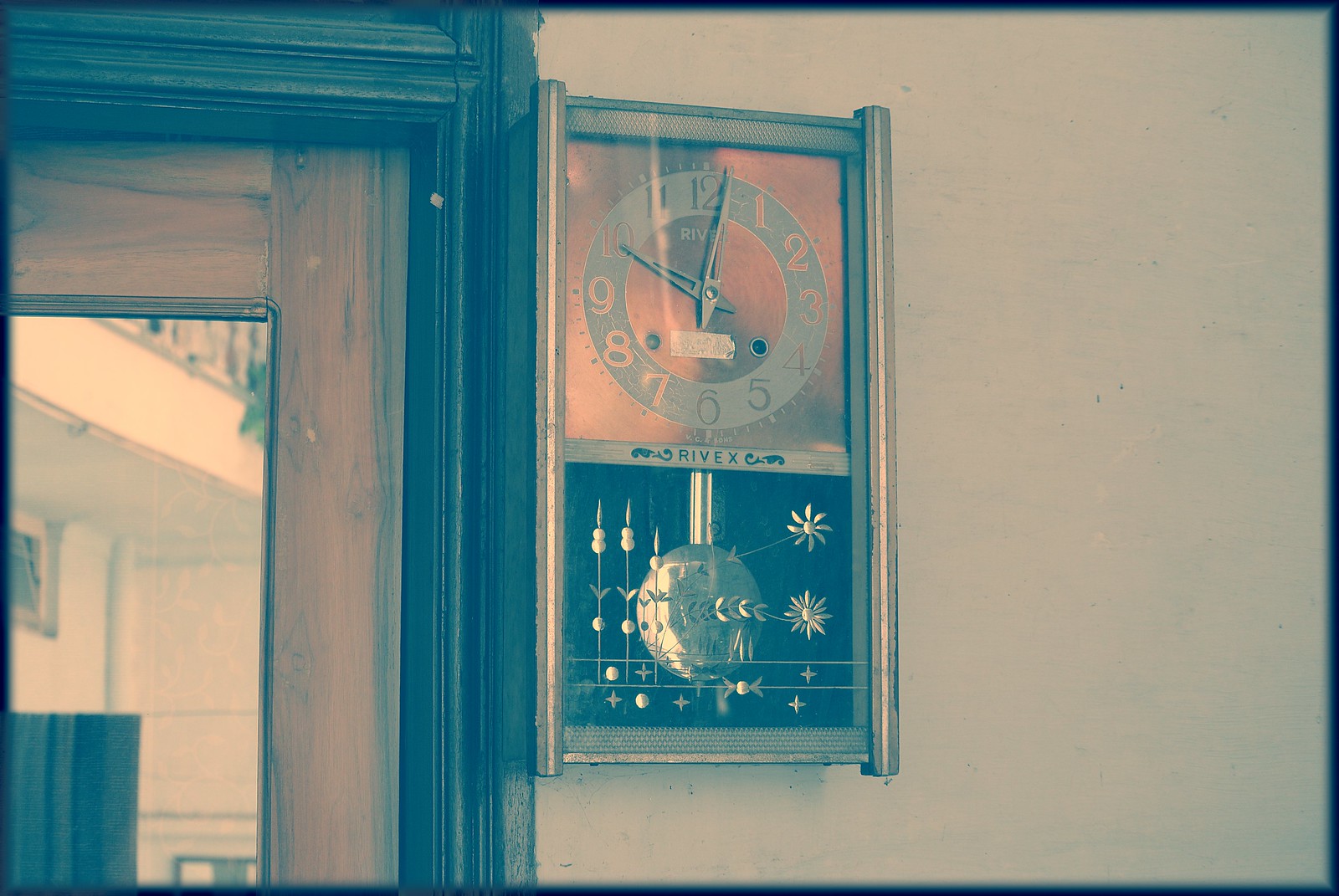This photograph, likely taken a few decades ago, captures a quaint interior scene. An off-white wall serves as the backdrop, adding a vintage appeal. To the left, a hefty wooden door with a black-framed glass panel offers a glimpse into the adjoining room, which features a visible second floor and a prominent banister. Adding a touch of classic elegance, a bronze wall-mounted grandfather clock is positioned to the right of the door. The clock's face is encased within a white circle displaying the numerals, while the striking gold pendulum swings gracefully behind a glass cover adorned with intricate golden designs. This well-composed image highlights the timeless charm of a bygone era.